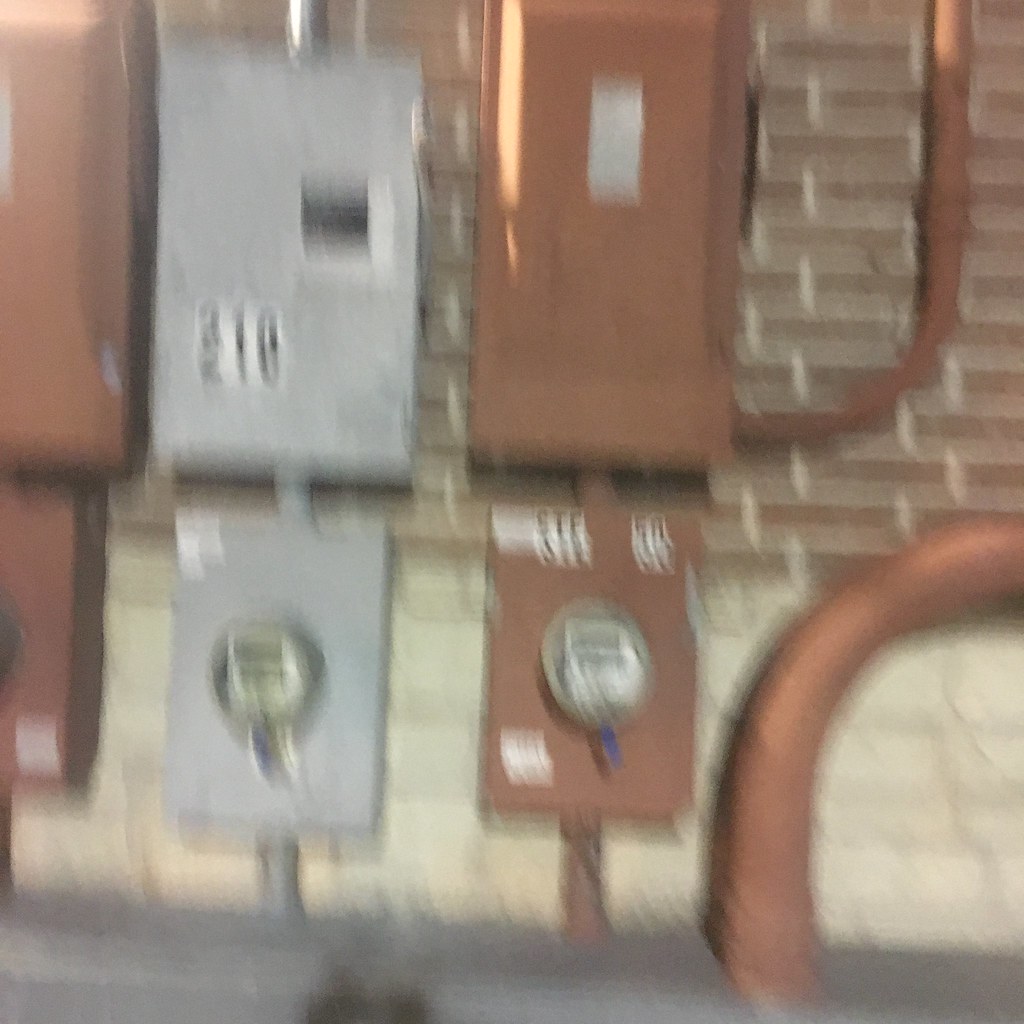A slightly blurry, square-shaped color photograph captures a red brick wall adorned with multiple electrical installations. The brick extends from the top of the image to almost the bottom, where it transitions into a yellow-painted section, indicative of a recent or intentional design choice. The ground at the base of the wall is faintly visible and appears to be a muted gray.

The lower right corner of the image features a bronze-colored light fixture, with its tube extending vertically downwards. On the wall, there are three prominently positioned electrical meter boxes. The meter boxes on the left and right sides are bronze, while the one in the center is gray. Each meter box has a corresponding pole that extends downwards to the floor and connects to another electrical box mounted directly above. Emerging from these boxes are matching metal tubes that ascend towards the ceiling, further emphasizing the structured chaos of urban infrastructure.